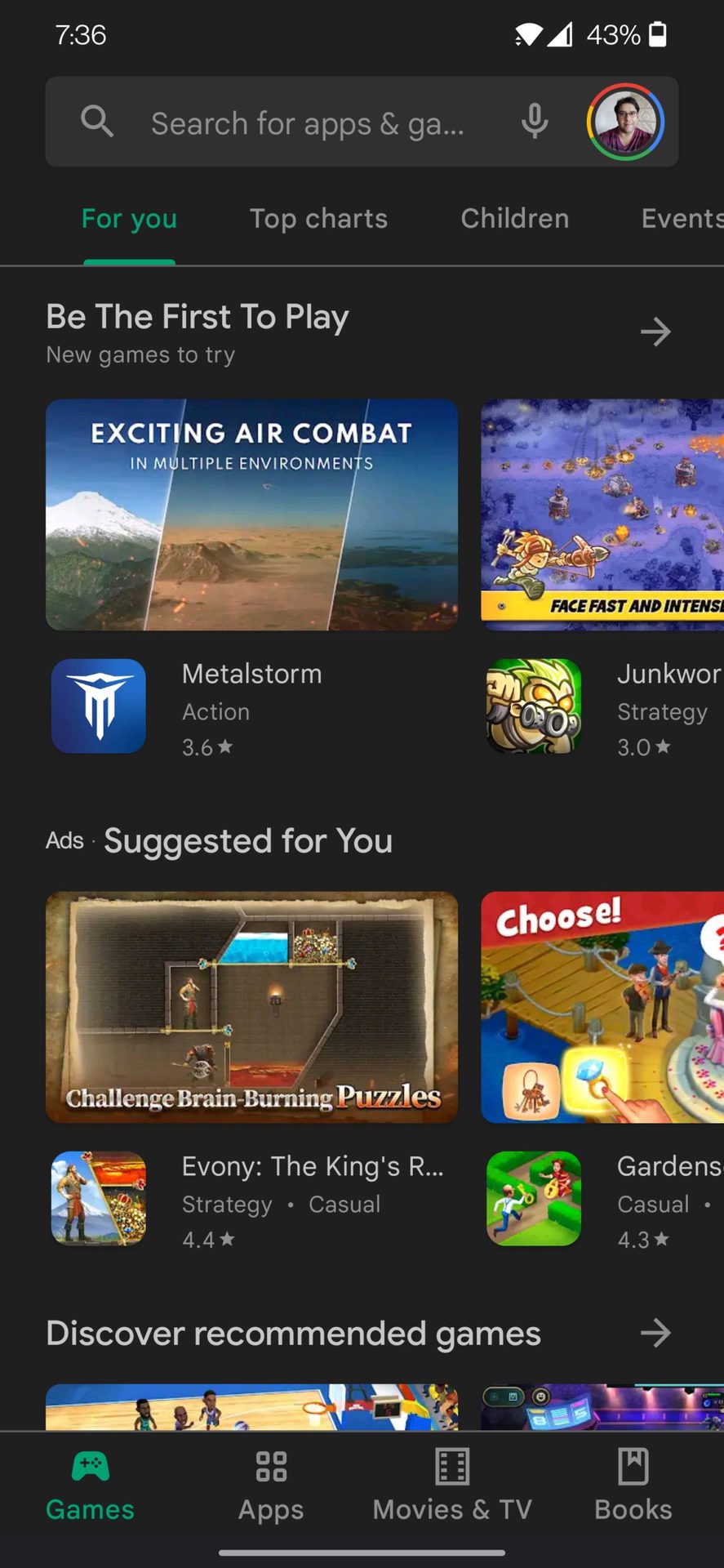The image showcases a smartphone screen displaying an app store interface. At the top, the status bar includes indicators for the time (7:36), battery percentage, and Wi-Fi signal strength. Beneath this, a search bar prompts the user to "search for apps and games," featuring a gray microphone icon for voice input. 

The screen's main section is divided into multiple colorful categories such as "For you," "Top charts," "Children," and "Events." A prominent banner invites users to "be the first to play new games," with the top-listed game being "Metal Storm." This action game boasts a 3.6-star rating and an engaging visual of a man in a purple shirt amid a vivid background featuring green, yellow, red, and blue hues. An accompanying image highlights "exciting air combat in multiple environments" like mountains, deserts, and water, denoted by a blue icon with a white logo.

Below, an ad section labeled "Suggested for you" showcases the game "Avani: The King's Rule," described as a strategy game involving "challenge brain-burning puzzles." Its displayed image features characters navigating through perilous settings with lava and water, and it holds a 4.4-star rating.

Further down, a section titled "Discover recommended games" presents a variety of other game suggestions, including an image resembling a basketball court. The entire interface is set against a gray background, providing a cohesive look.